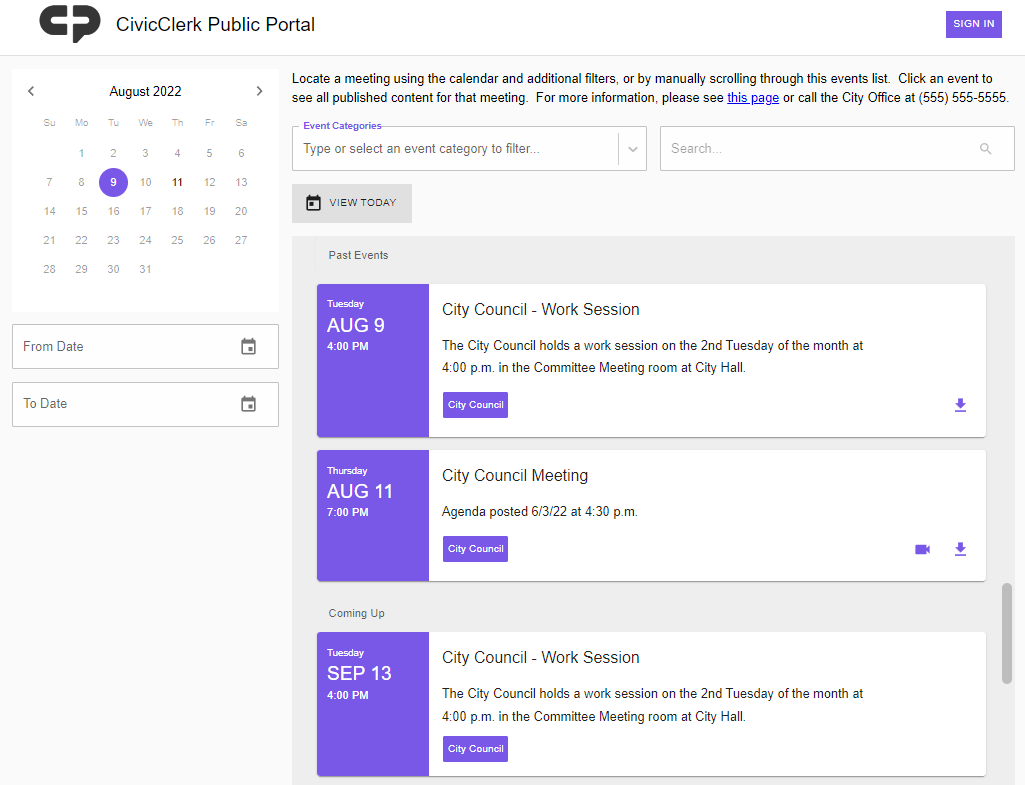This image captures an online portal interface, specifically the Civic Clerk Public Portal. The portal appears square in shape, though it lacks defined borders. At the top center of the page, there's a distinctive logo resembling a horizontally elongated "Q," bisected by a white bar. Adjacent to this logo, the title "Civic Clerk Public Portal" is displayed in black font.

In the top right corner of the interface, there is a horizontally oriented purple rectangle housing a white sign-in button. Running along the top of the portal is a thin gray border featuring a calendar icon, which is a simple square graphic. This calendar is currently set to August 2022, with the 9th highlighted by a purple circle and white text. Navigation arrows flanking the calendar allow for month selection changes, and there are fields below to input dates manually.

To the right of this calendar section, a box with black text instructs users to "locate a meeting using a calendar and additional filters or manually," followed by a filtered list of results. Below this section, there is a gray box labeled "view today" in black font, listing upcoming events. 

The first listed event is for August 9th and is marked by a purple box with white text, alongside a white box with the black text "City Council." The next event, dated Thursday, August 11th, shares the same City Council labels. Following these, an upcoming event is scheduled for September 13th at 4 p.m., clearly indicated as a "City Council Work Session."

The layout and organization of this portal are designed to provide users with an intuitive way to locate and manage civic meetings and related events efficiently.